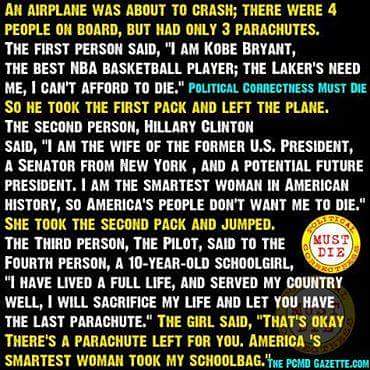The image features a black backdrop with yellow, white, and blue text that reads: "Political correctness must die," accompanied by a logo. In the bottom right-hand corner, it states "PCMDGazette.com." The content is a satirical joke involving an airplane crisis. There are four passengers but only three parachutes. The first person, Kobe Bryant, claims his necessity for survival due to his status as the best NBA player and it highlights in blue text "political correctness must die" as he takes a parachute and jumps. The second, Hillary Clinton, boldly proclaims her crucial political roles and self-declared intelligence, then grabs what she believes is a parachute and jumps. This leaves the pilot offering the last parachute to a 10-year-old girl. The punchline reveals that the young girl, with astute observation, tells the pilot not to worry because America's "smartest" woman mistakenly took her school bag instead of a parachute, implying there are still two parachutes left.